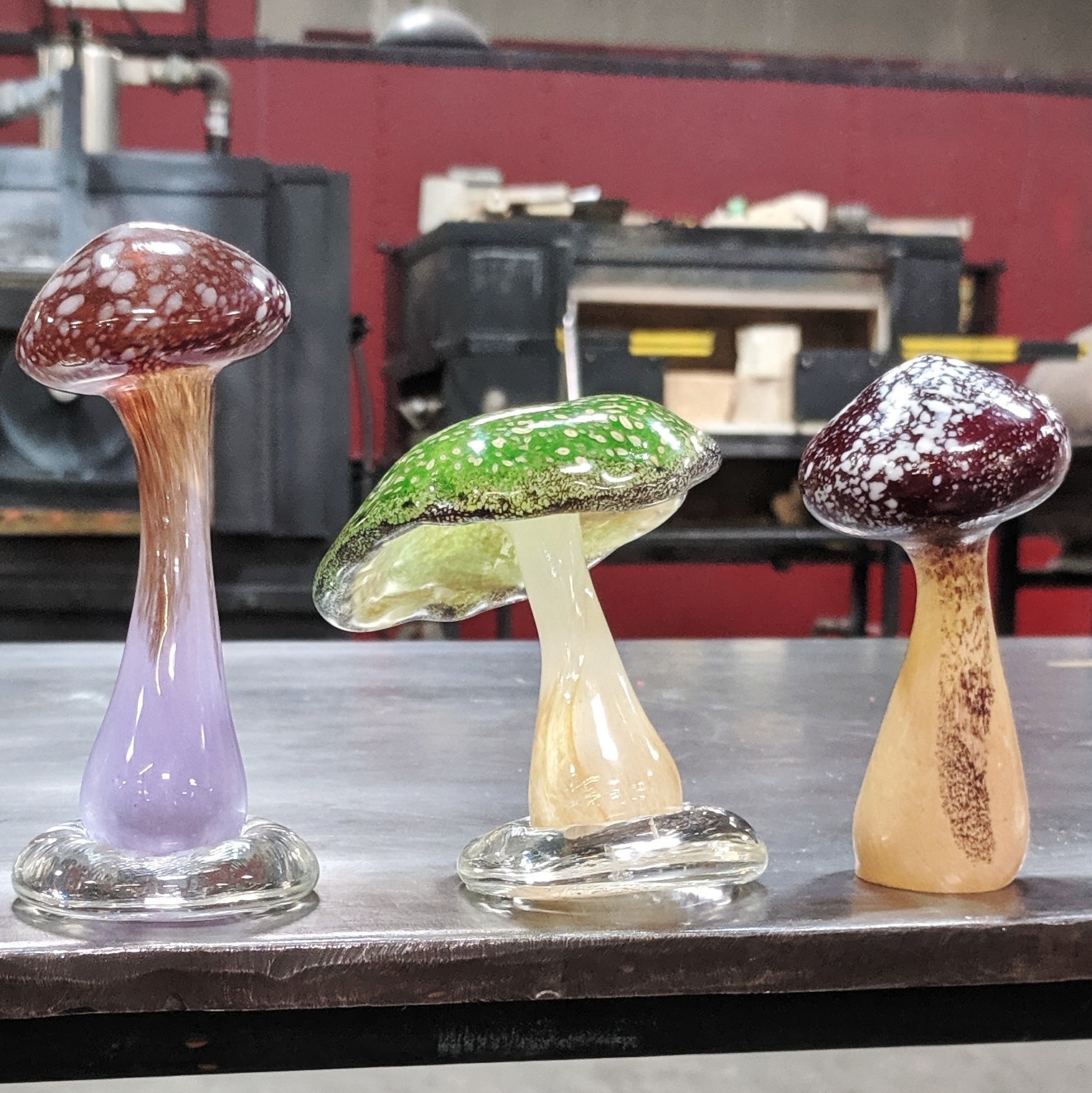In this detailed image, three exquisite blown glass mushroom figurines are showcased on a black table. Each mushroom varies in height, color, and form. The mushroom on the left side is the tallest and has a slender structure, sporting a distinctive red cap adorned with white blotchy spots. Its stem transitions from a foggy blue at the base to an off-white hue as it meets the cap. The middle mushroom is the shortest and widest, featuring a vibrant green cap also adorned with white speckles. Its robust stem starts with a clear base, shifting to a cream tan color and then to an off-white as it nears the cap. The rightmost mushroom, medium in height, boasts a dark burgundy cap with large white blotches. Its stem is a mix of orange and maroon shades and is wider at the base. In the background, elements of machinery are visible, adding contrast to the artistic display.